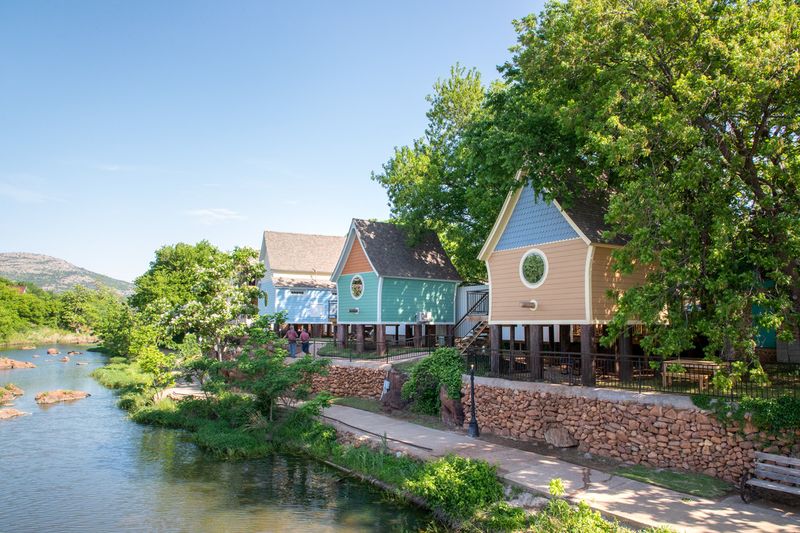The image depicts a tranquil lakeside scene with three uniquely designed houses perched on wooden stilts, giving them the appearance of oversized birdhouses. Each house features a large circular window resembling the "entrance" of a birdhouse, complemented by a triangular, A-shaped roof. The houses are painted in vibrant hues: the nearest house has a beige center with a blue roof, the second features a turquoise center with an orange and black roof, and the third, more distant house appears light blue.

These structures are situated along a sidewalk that meanders by a peaceful lake, surrounded by abundant greenery and large rock formations. The water near the shoreline is shallow and becomes darker and bluer as it extends towards the horizon. Two people are seen standing near a fence beside the sidewalk, one wearing a red top and dark jeans, and the other in similarly dark attire. 

In the lower right corner of the image, there is a silver and gray wooden bench. The scene is further accentuated by a mountainous hill range in the background and various other benches and white buildings visible in the distance. The first house, supported by gray wooden stilts, stands among lush bushes and trees, with a foundation of tan brown stonework.